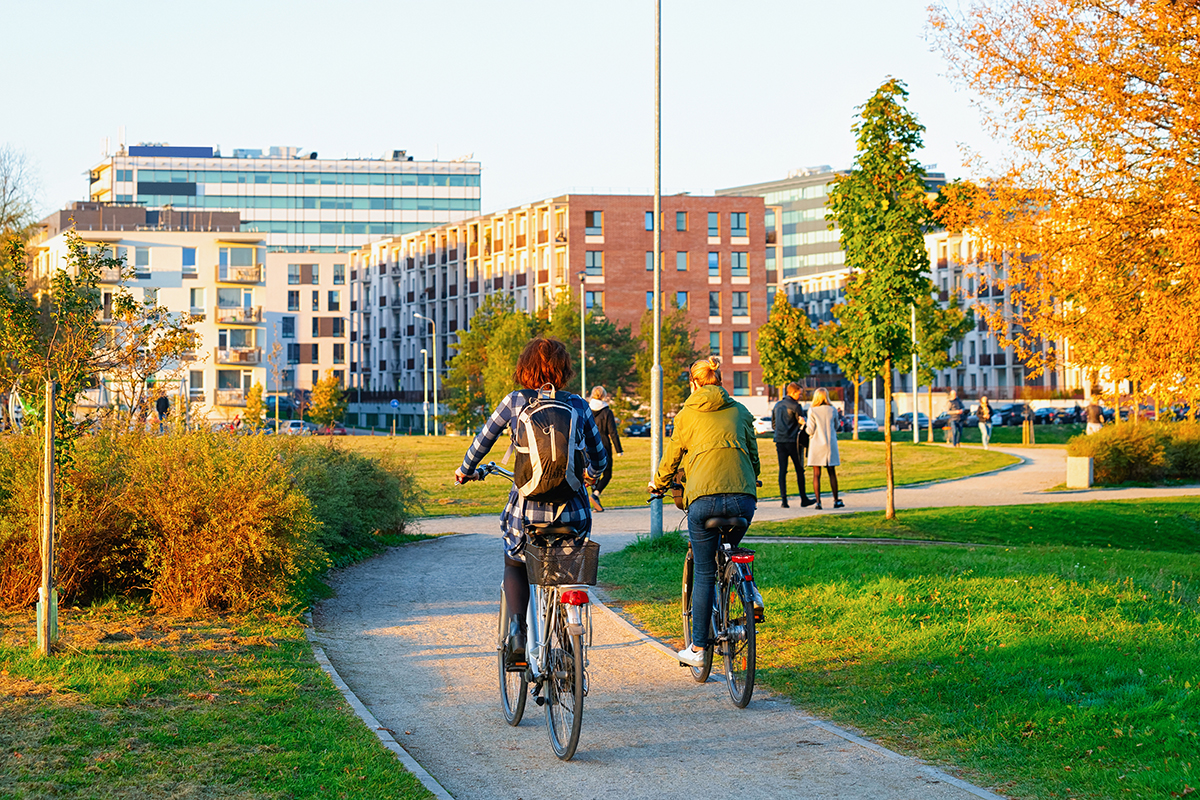In this vibrant urban scene, a photograph captures a lively moment in what appears to be a well-kept park or university campus. The setting showcases a smooth asphalt bike path flanked by lush, green grass and dotted with shrubs, small trees, and a striking yellow-leafed tree hinting at autumn. The path, which gracefully snakes through the park, is teeming with activity. Central to the image are two women on bicycles: one with red hair, dressed in a plaid shirt and sporting a black and white backpack atop her bike's rear basket, and another in a green jacket and blue jeans. Both are riding side by side, exuding an air of casual enjoyment. They are followed by two people walking along the path: a man and a woman. The scene is illuminated by bright, possibly early evening sunlight, casting a warm, inviting light across the entire scenario, while the sky above appears unusually white due to the photograph's exposure. In the background, several multi-story buildings, possibly apartment complexes or dormitories, further emphasize the urban nature of this bustling and scenic environment.